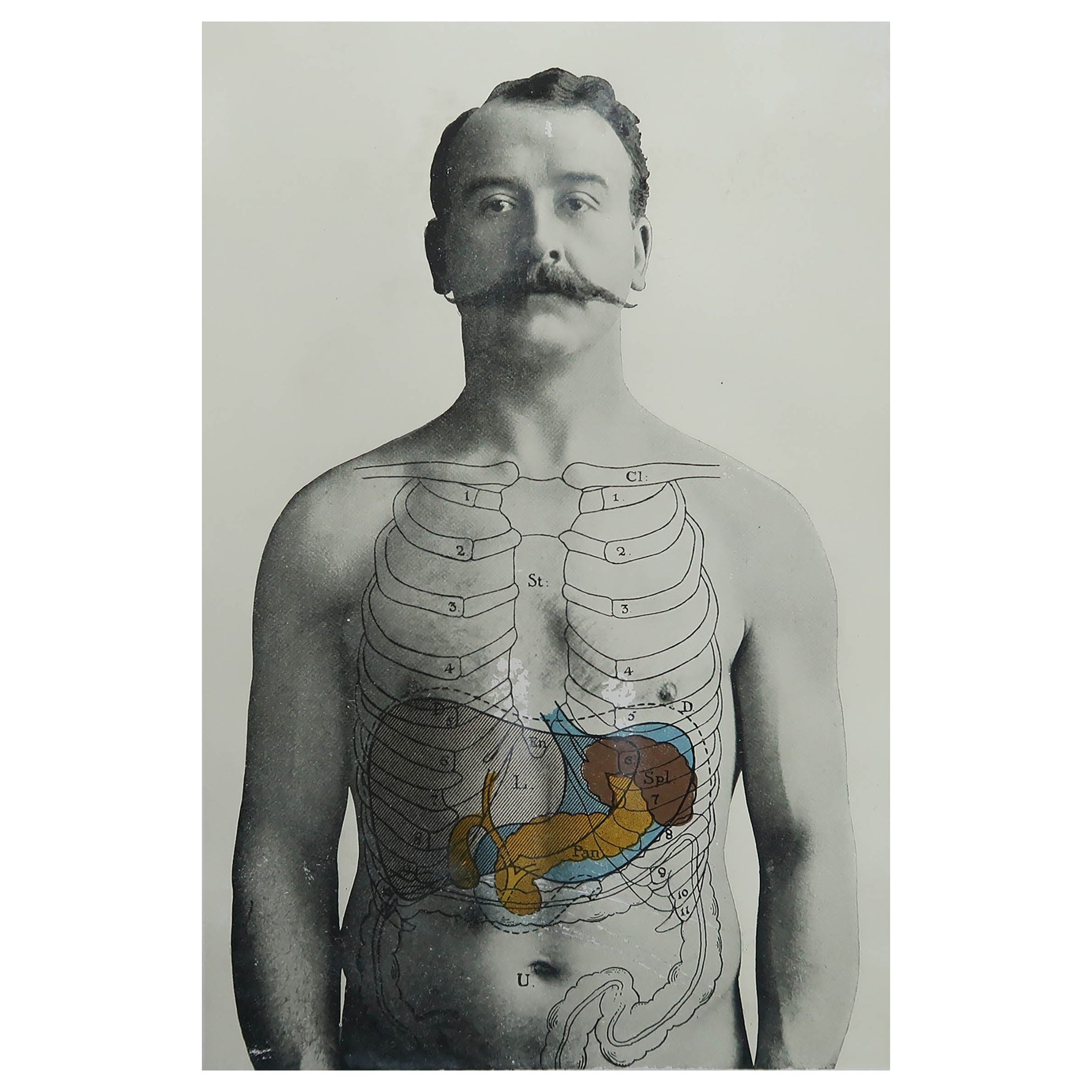This is a black and white photograph, likely taken in the 1920s or 1930s, depicting a shirtless Caucasian man with distinctive facial features and anatomical drawings on his chest. The man has short, dark brown hair that is parted on the side and slightly wavy, and he sports a long, elaborate mustache that extends horizontally beyond his jawline. The photograph, which measures approximately five inches high and three inches wide, captures the man from his head down to just below his hips, making it unclear whether he is wearing any pants.

The most striking element of the photograph is the detailed anatomical illustration overlaid on the man's chest. This drawing includes his skeletal system, with his clavicle and rib cage prominently labeled and numbered. The internal organs are also depicted and labeled: the spleen is colored dark brown and marked "SPL," the pancreas is a mustard yellow labeled "PAN," the liver is dark gray labeled "L," and the stomach is a distinctive light blue. The background of the photograph is a light gray, providing a stark contrast to the intricate and colorful anatomical details. This unique image blends elements of medical illustration with early 20th-century portrait photography, creating a fascinating visual study.